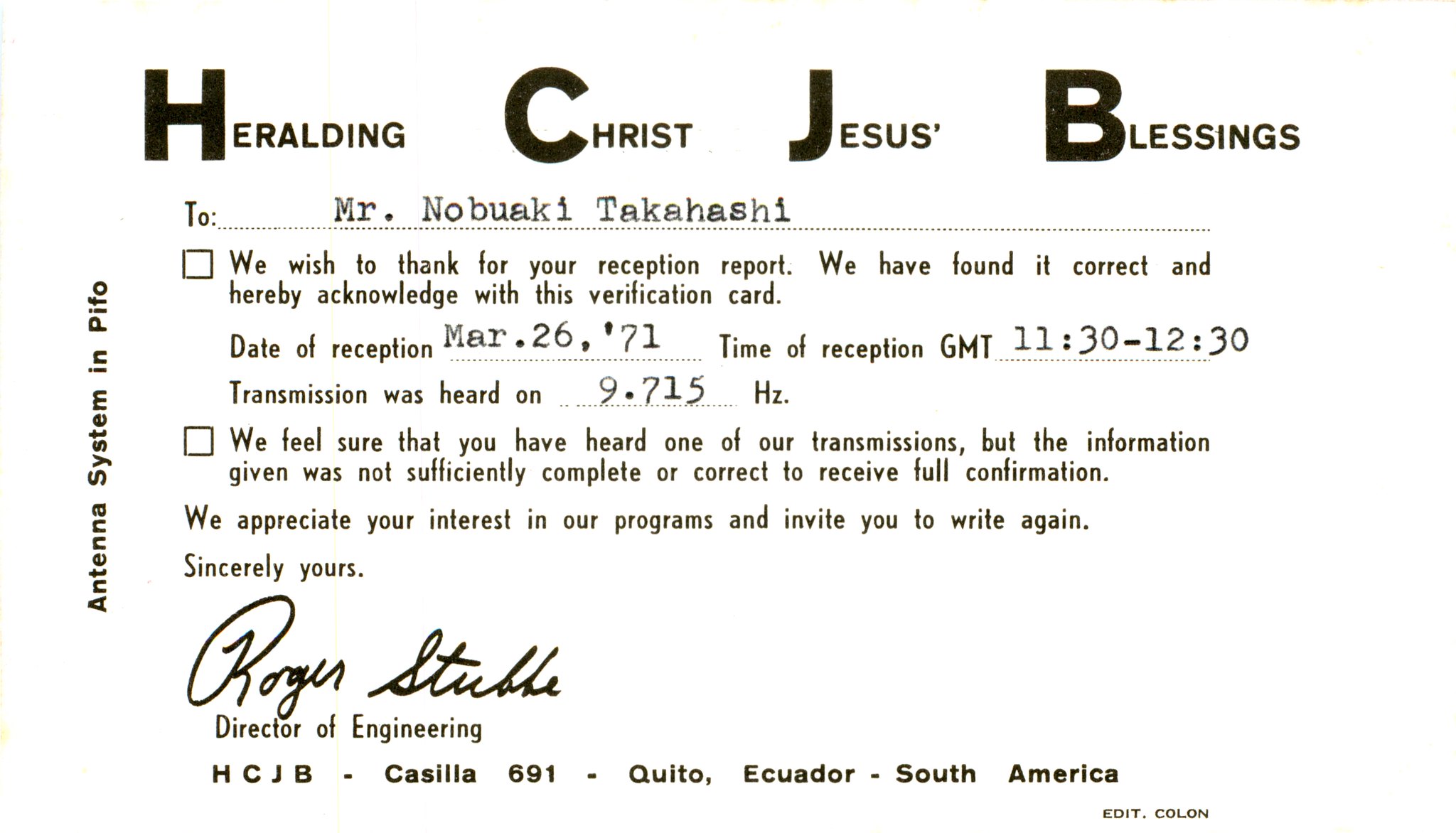The image depicts an old scanned document resembling a postcard. At the top, bold and prominently capitalized letters spell out "Heralding Christ Jesus Blessings," with each word's initial letter being significantly larger and emphasized—H, C, J, B. Below this heading, the document is addressed to Mr. Nobaki Takahashi and expresses gratitude for a reception report. It acknowledges the reception on March 26, 1971, with the specific time of 11:30-12:30 GMT, and the transmission frequency of 9.715 Hz. There are areas that mention checkboxes and the contents indicate it relates to radio transmissions. The document also contains detailed breakdowns and numbers explaining the report and specifies that the information provided was not complete enough for full confirmation, but appreciation for the interest in the programs is noted. It is signed by Roger Stubble, the Director of Engineering, and originates from HCJB Casilla 691, Quito, Ecuador, South America.